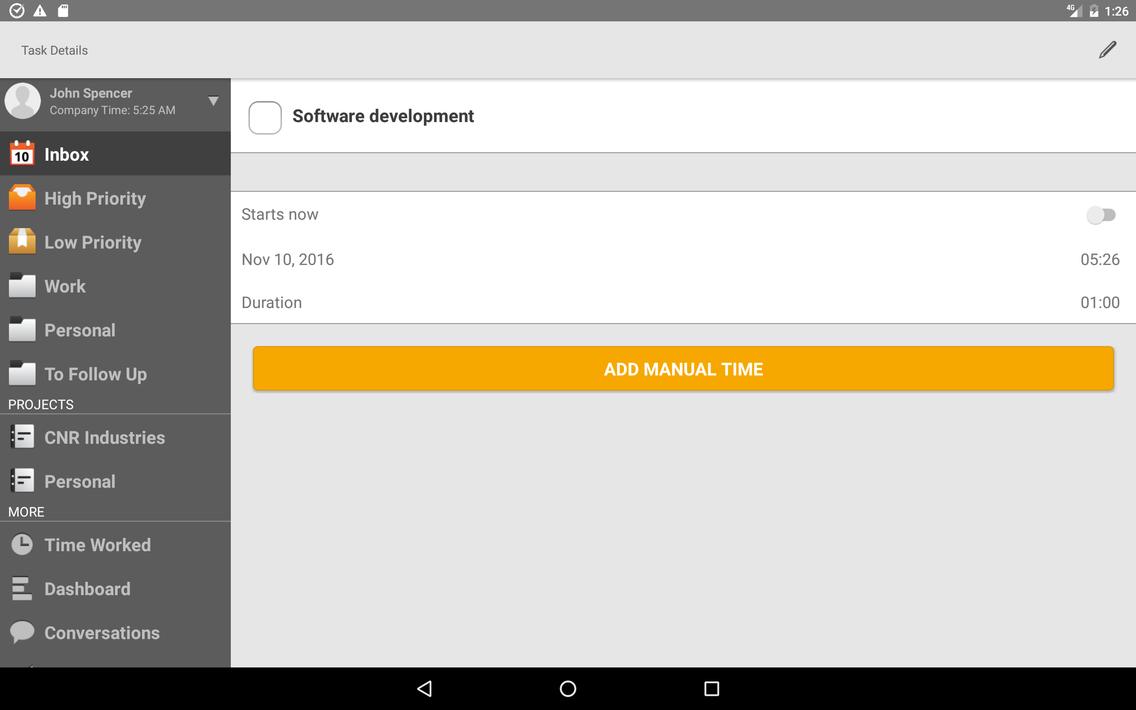In the image, the top left corner features a grey triangle and a battery icon displaying 1.6%. Beneath it, there are chat details with a pen icon, listing "John Spencer" and the company type. The time "5:25 AM" is shown next to a dark grey rectangle labeled "calendar" and "inbox." Within the inbox section, there are priority indicators: an orange one for "high priority" and another for "low priority." Below these, there are folders marked "work," "personal," and "to follow up on products."

Further down, there is a clock showing a specific time, paired with a dashboard icon and a speech bubble labeled "conversations." Additionally, there's a grey rectangle indicating an event that occurred just now, with a time stamp of "November 10th, 2016, 05:26," and a duration of "01:00." A yellow rectangle highlights an option to "add manual time," with "now" written in white text at the center. 

Toward the bottom, a black bar spans the width of the image. A series of icons—including a high-waisted triangle, a circle, and a square—are present. The overall layout presents various elements related to software development, personal and professional organization, and real-time communication.

The different shapes and colors suggest an interface with multiple functionalities and notifications designed to manage tasks, time, and communication efficiently.